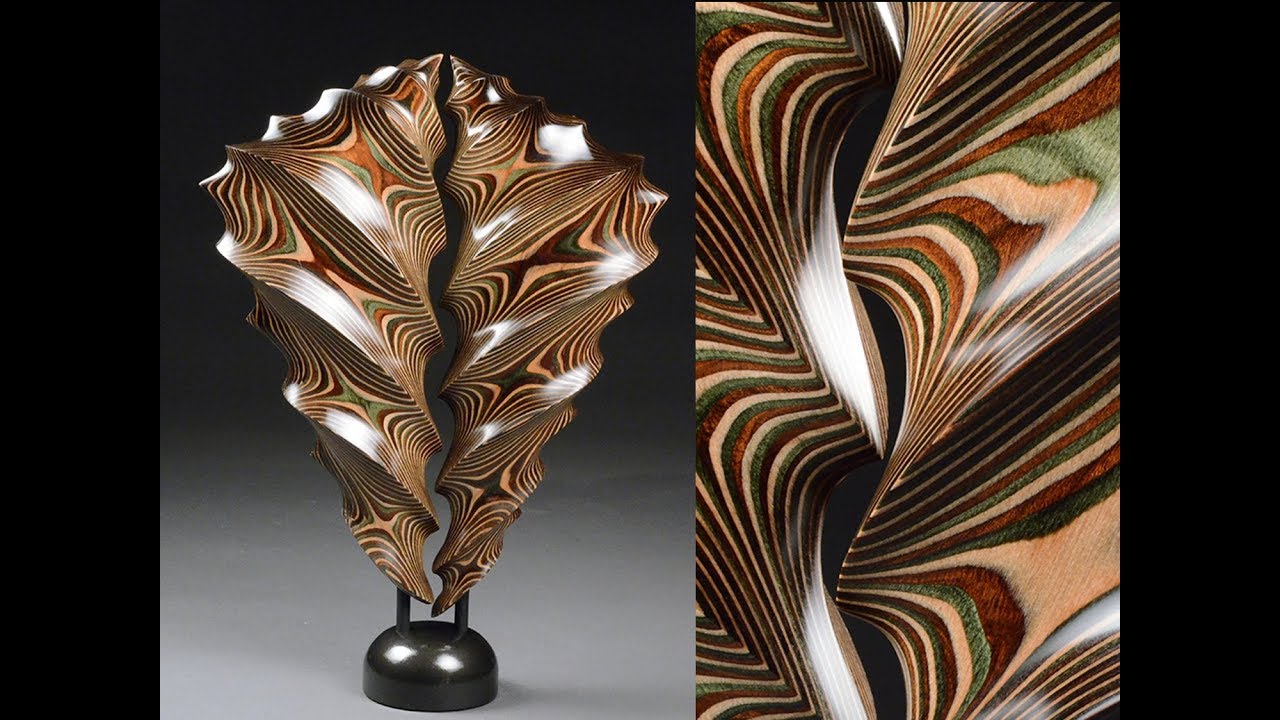The image features two color photographs of a wooden sculpture, displayed side-by-side against a solid dark black rectangular background with vertical black bars on either side. The photograph on the left captures the entire sculpture, while the photograph on the right presents a detailed close-up. The sculpture itself consists of two wavy, seashell-like pieces resembling inverted cones or butterfly wings, intricately carved with swirling patterns and mounted on a black, dome-shaped metal base. Each piece is supported by thin metal rods extending from the base. The sculpture's wood shows visible grain, with a mix of natural brown hues, stained portions, and inlaid stripes in shades of green and red, displaying a shiny finish. The close-up on the right emphasizes the detailed wood grain and the intricate, multi-colored inlay, highlighting the craftsmanship and texture of the piece.